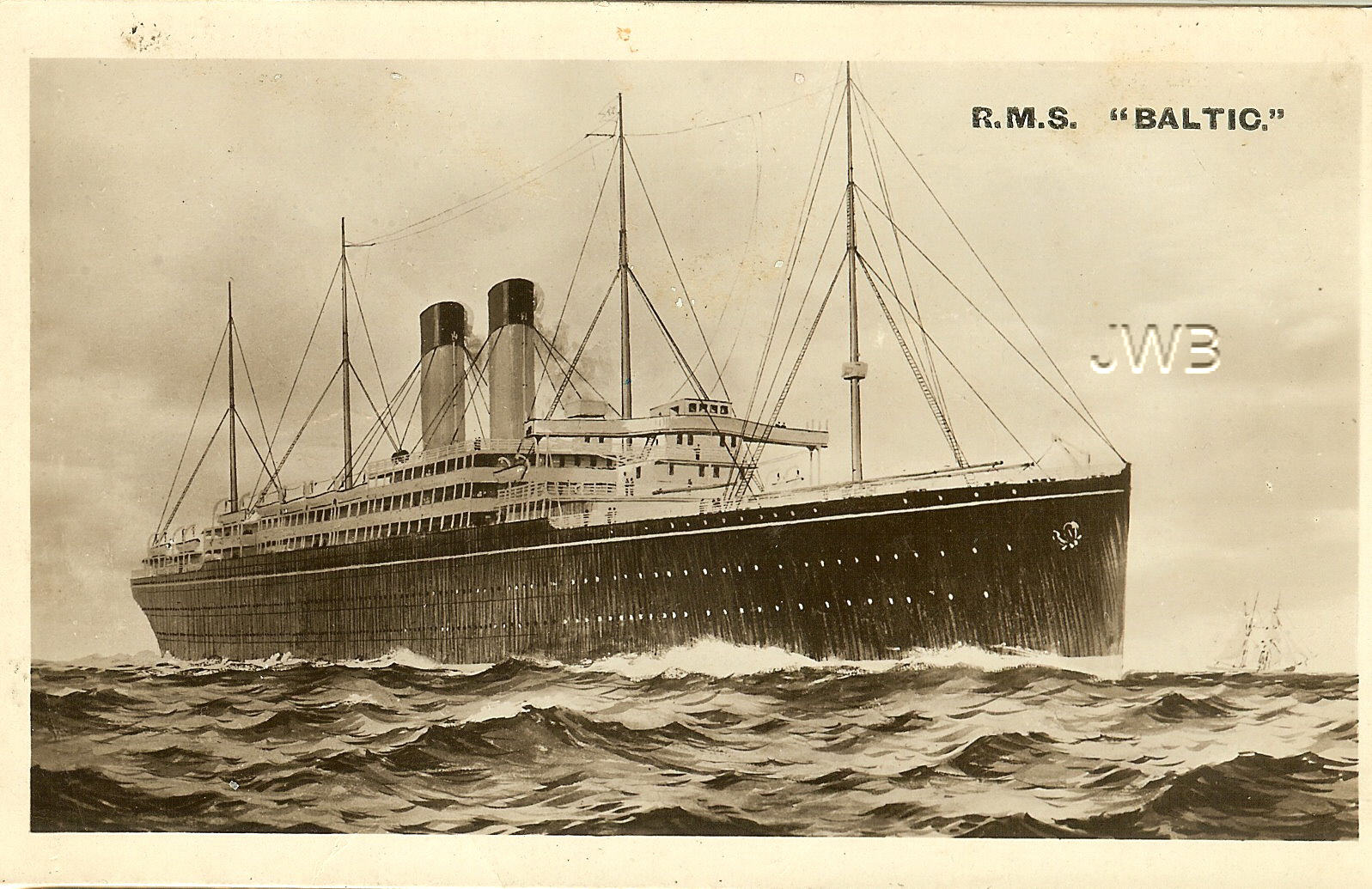This is an old, black-and-white illustration of the RMS Baltic, appearing worn and water-stained with a pinkish hue along the borders. The ship's name, "R.M.S. 'Baltic'.", is inscribed at the top right corner, alongside the imprint "JWB." The artwork, likely done in pencil or charcoal, showcases the colossal steamship navigating a gray, choppy sea under a cloudy sky. The vessel features four masts, multiple decks both above and below with numerous windows, and two prominent smokestacks in the center. The ship's riggings, poles, and wires are meticulously detailed, emphasizing its grand, industrial scale.